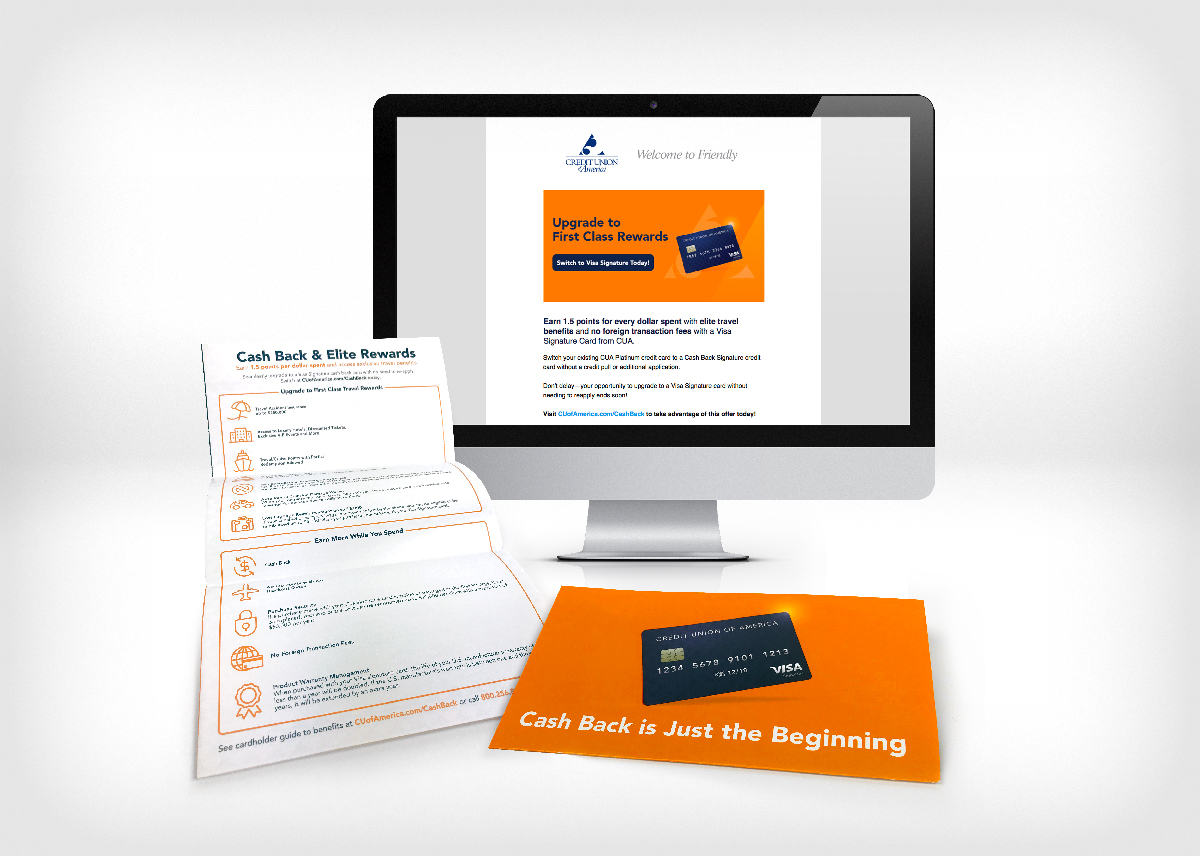The image features a modern, silver-finished PC with a black-bordered screen displaying a web page. The web page prominently features an 8x10 document with the company's logo at the top, followed by text that reads "Welcome to" possibly "Friendly," and an orange rectangle highlighting "Upgrade to First-Class Rewards" in black font. Below this, a small bar and an icon of a credit card can be seen, alongside extensive small print detailing the rewards, such as "Earn 1.5 points for every dollar."

To the left of the PC, there are printed-out pages arranged neatly on a flat surface. These pages bear the titles "Cash Back" and "Elite Rewards." Another visible slogan on the surface remarks, "Cash Back is Just the Beginning," emphasizing the benefits of the credit card. The credit card itself is also displayed, adding a visual reference to the web page content and printed materials.

The PC is supported by a modern, curved pyramid stand, completing the sleek and organized theme of the setup.